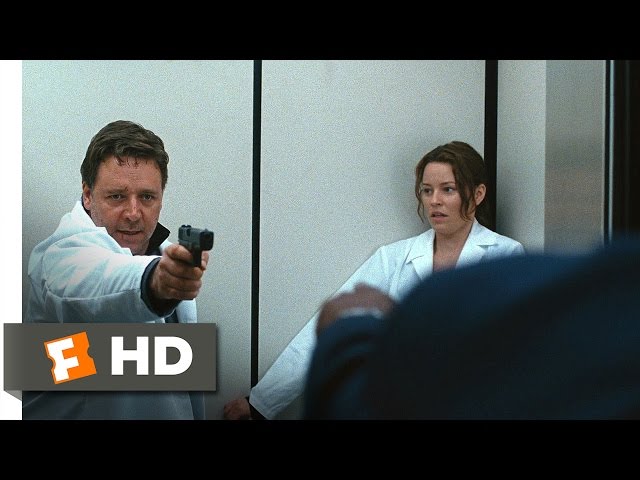The image is a still from a movie, possibly featuring Gerard Butler and Elizabeth Banks, and appears to be framed as a thumbnail from a YouTube video or movie website, with black bars lining the top and bottom. The setting is an elevator. Gerard Butler's character, positioned on the left, is dressed in a white lab coat, possibly masquerading as a doctor. He holds a gun in his right hand, pointing it with intense determination at an unseen man in a blue suit, of whom only a shoulder and hand are visible. There is a cut on Gerard's lip, adding to the tension in the scene. In the right corner, Elizabeth Banks' character, also clad in a white lab coat, cowers fearfully against the elevator's wall. Her right arm is outstretched against the wall, and her wide eyes are fixed on Gerard, reflecting her trepidation. At the bottom of the image, a Fandango label indicating "HD" can be seen.